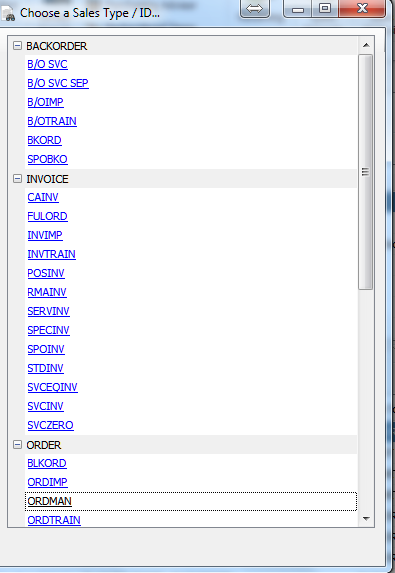This image, presented in portrait mode, appears to be a screenshot taken from a mobile phone. The background features a light blue color scheme. Positioned in the upper left corner, there is an icon resembling a piece of paper alongside a pair of binoculars, accompanied by the text "Choose a sales type/ID..." followed by ellipses.

Across the top of the screen are four buttons: 
1. A double-sided arrow symbolizing sort or navigation.
2. A minimize button.
3. A full-screen button.
4. A red 'X' button for closing the window.

The main content area displays a list of terms, seemingly related to sales types or inventory actions:
- Backorder (highlighted)
- B/O Services
- B/O Services SEP
- B/O IMP
- B/O Train
- BKORD
- SPOBKO
- Invoice (also highlighted)
- Kainv
- Fulord
- Invimp
- Invitrain
- Pause
- Inv
- RMAINV
- Servinv
- Spessinv
- Sporinv

Next, another highlighted term reads "Order," with related terms below:
- BLKORD
- ORDI
- IMP
- ORDMAN (underlined and surrounded by dots)

These terms appear to be live links or buttons likely designed to open corresponding documents or sections within a sales or inventory management application.